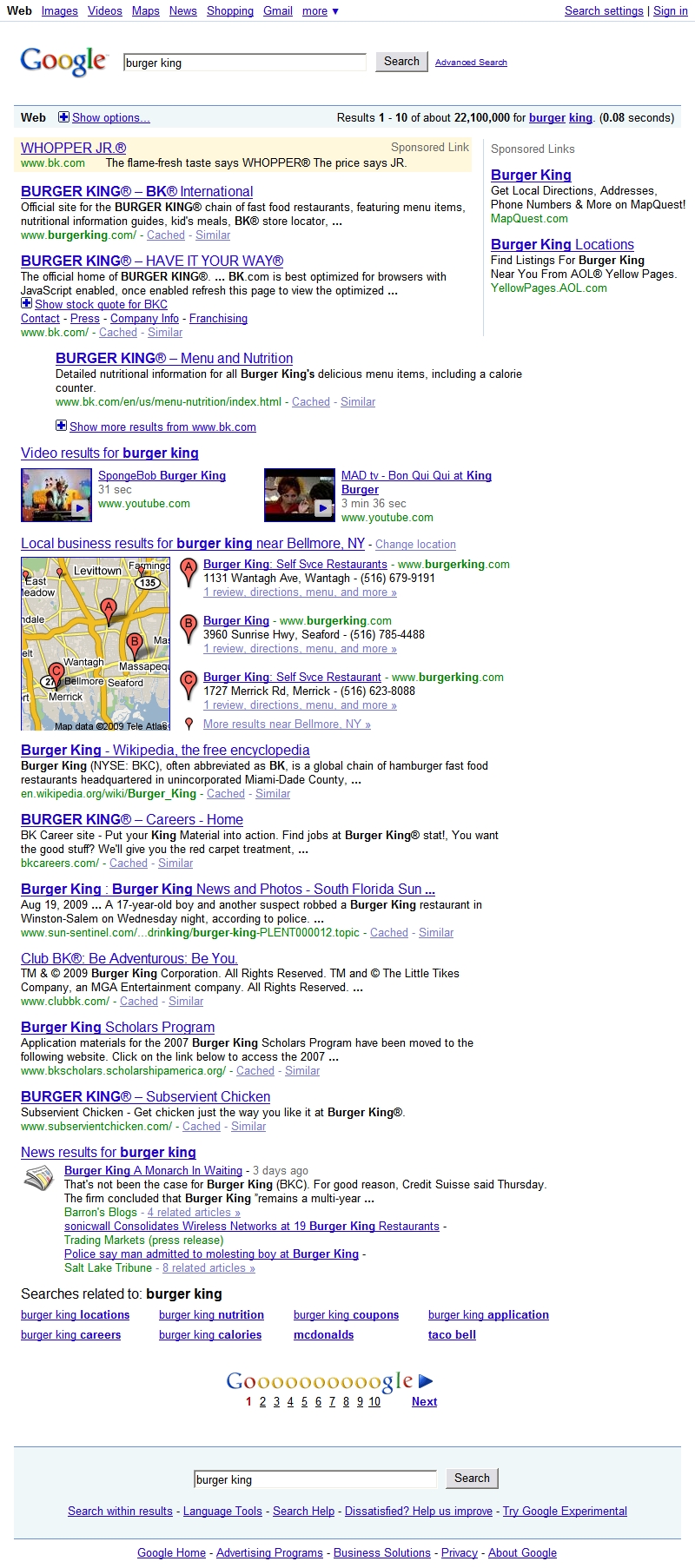The screenshot captures a Google search results page for the query "Burger King." The layout features a crisp white background with blue font for the navigation links at the top, which include categories like Web, Images, Videos, News, Shopping, and Gmail. The 'Web' category is currently selected, indicated by its different appearance. On the top right corner, there are options for 'Search settings' and 'Sign in.'

Just below the navigation menu, the multicolored Google logo is prominently displayed above a search bar where "Burger King" has been entered. The search button to execute the query is located to the right of the search bar and is gray in color.

As you move down the page, the search results are displayed in descending order, blending text and images. The top result is labeled "Burger King," marked as the official site, followed by additional descriptive text. Various search elements are present, including embedded videos with thumbnails and a map highlighting different Burger King locations. The map is shaded in blues, greens, and yellows, with red markers pinpointing the exact locations.

At the bottom of the page, there's a playful rendition of the word 'Google,' stretched to include multiple 'O's, indicating paginated search results.